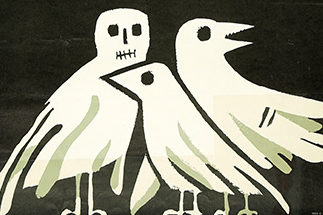This is a detailed drawn or computer-generated image featuring three distinct birds set against a black background. The smallest bird is depicted with a closed beak, looking to the left, showcasing a solitary black eye. Its feather colors are predominantly green and white. The second largest bird is oriented to the right with its mouth open, revealing jagged shapes that resemble teeth. It shares the same green and white feather coloration. The largest bird faces directly forward, its mouth depicted as a straight line with vertical slashes, giving it an appearance similar to a cut. This bird has large, square eyes and a simple black line for a nose, with the same green and white feather palette. The black background accentuates the vivid colors and distinct features of the three birds.